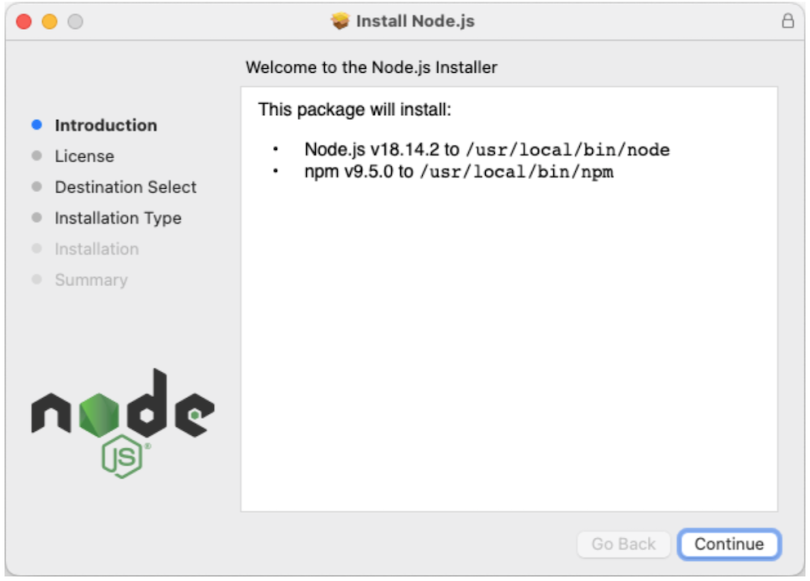The image showcases a gray rectangular interface with curved corners, accentuated by a darker gray outline. In the top left corner, three dots appear in succession: red, yellow, and gray. Along the top edge, from left to right, there is an icon of an opened cardboard box accompanied by the gray text "Install Node.js," followed by a lock icon outlined in gray positioned at the top right.

On the left side of the interface, there are six dots aligned vertically. The top dot is blue, and the remaining five dots are in shades of gray that gradually become lighter towards the bottom. The gray shades shift from a darker gray for the three dots immediately under the blue dot to a lighter gray for the final two dots.

The topmost option, indicated by the blue dot, features bold black text reading "Introduction." Below this section of text, the Node.js logo is displayed, with the "N," "G" and "E" in black and the "O" rendered as a rotated green hexagon. Beneath this logo, there is another green hexagon outline containing the letters "JS" inside it.

Positioned at the bottom right of the interface is a "Continue" button, which is outlined in blue, providing a clear call to action.